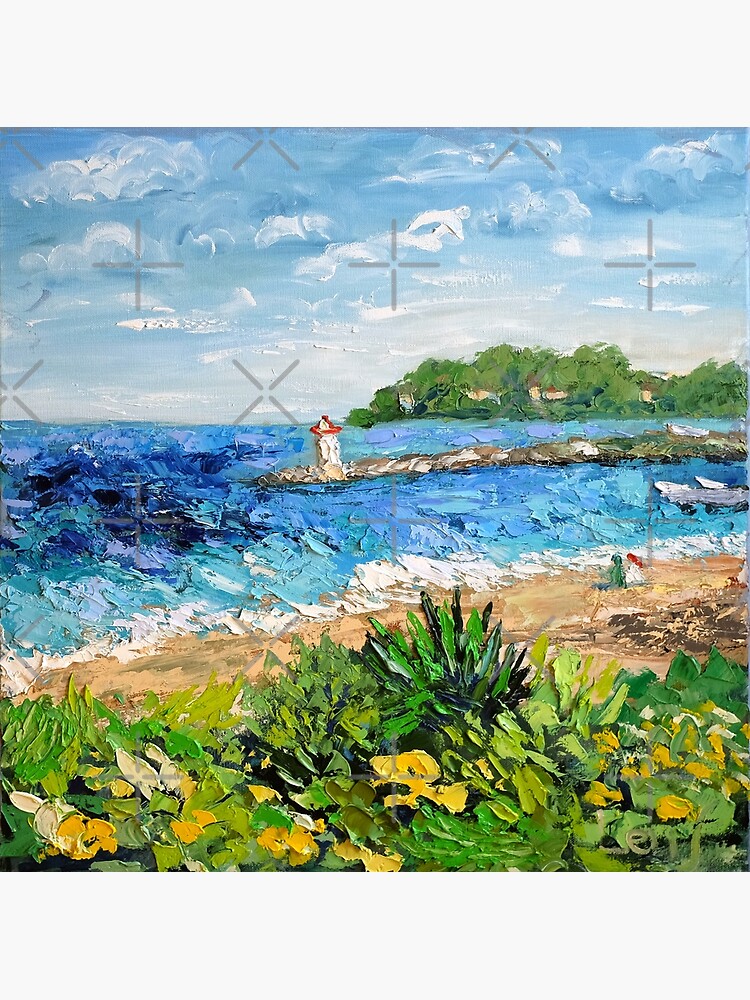The image is a portrait-oriented photograph featuring a square painting with an off-white border at the top and bottom. The painting presents an outdoor seaside scene done in very thick, chunky strokes of paint, giving it an abstract quality. Starting from the foreground, there is a grass-covered area with yellow flowers or leaves. Just beyond this grass, a sandy beach extends across the lower part of the scene. 

On the beach, towards the right side, there are two abstract figures; one is painted green, and the other is in white with either a red hat or red hair, seated possibly near some rocks. Where the beach meets the water, the sea is depicted with shades of blue interspersed with white to indicate waves. Off in the distance, a strip of land juts out into the sea, hosting a distinct white and red lighthouse.

Further back, mountainous forms rise beneath a sky filled with scattered puffy white clouds against a blue backdrop. The overall painting also has a unique feature: a grey cross, composed of four sticks, overlays the entire scene, adding to its abstract and textured appearance.